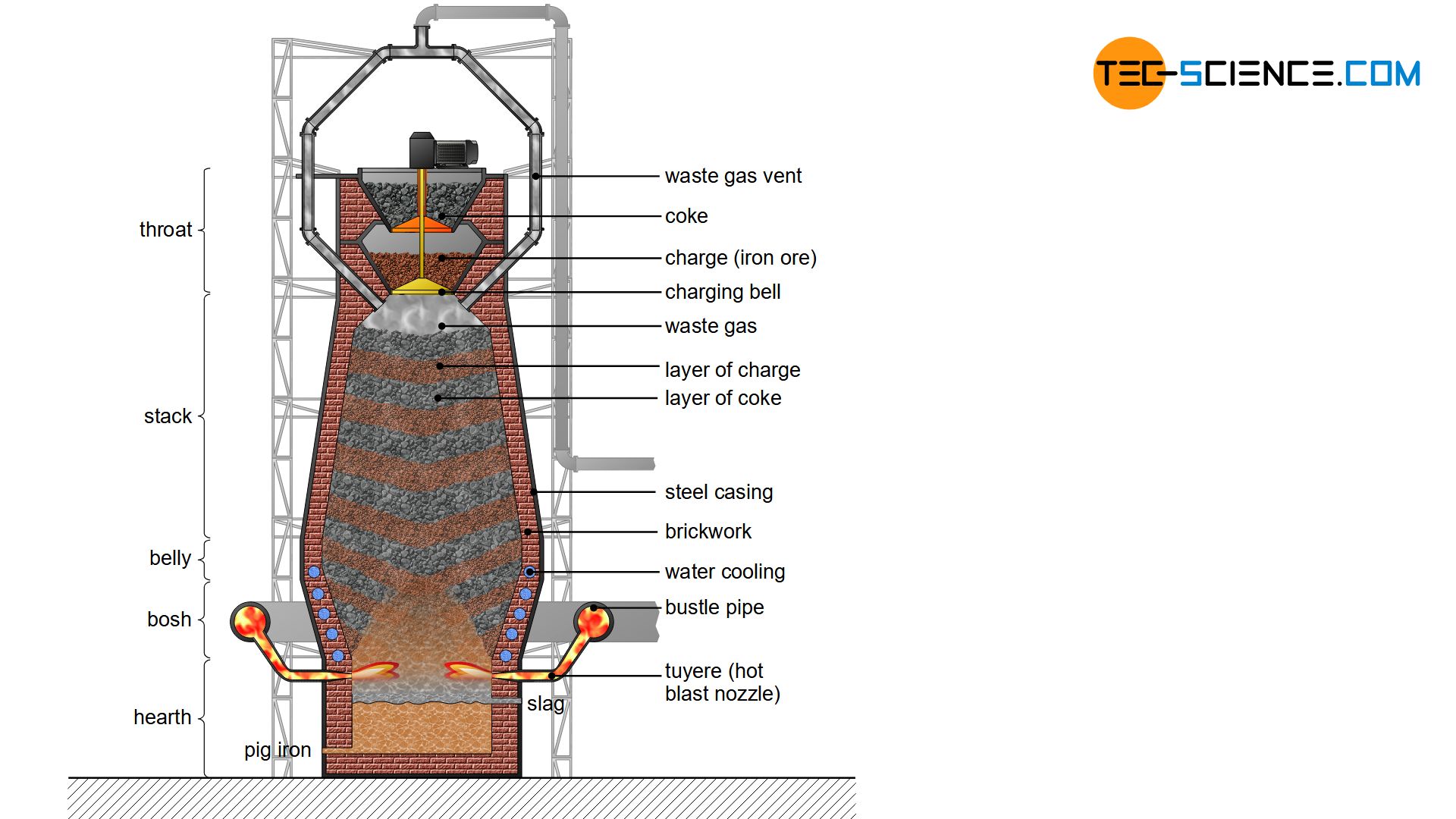This image is a detailed cutaway side view diagram of a blast furnace, which is used to melt iron ore into its various components. The furnace is primarily constructed with red brick and shows a brown, squarish base that curves outwards and then inwards as it ascends. The structure includes gray and brownish-red stripes in the middle, with yellow and red elements extending from the sides. The top features two partial triangles, one gray with orange accents and one brown with yellow accents, indicating different materials or sections. A complex scaffold-like structure sits above the furnace.

The diagram labels components from bottom to top on the left side as hearth, bosh, belly, stack, and throat, highlighting key areas within the furnace. On the right side, the labels include waste gas vent, coke, charge iron ore, charging bell, waste gases, layers of charge and coke, steel casing, brick work, water cooling, and bustle pipe, indicating the inputs and outputs of the process as well as structural elements. The bottom of the tower design also shows where pig iron and slag are collected. Surrounding the furnace are various pipes and apparatuses, which direct waste gases and provide hot blasts necessary for the furnace operation. The entire diagram emphasizes the internal and external structure required to maintain the system and the separation process. This detailed illustration is by tech-science.com.